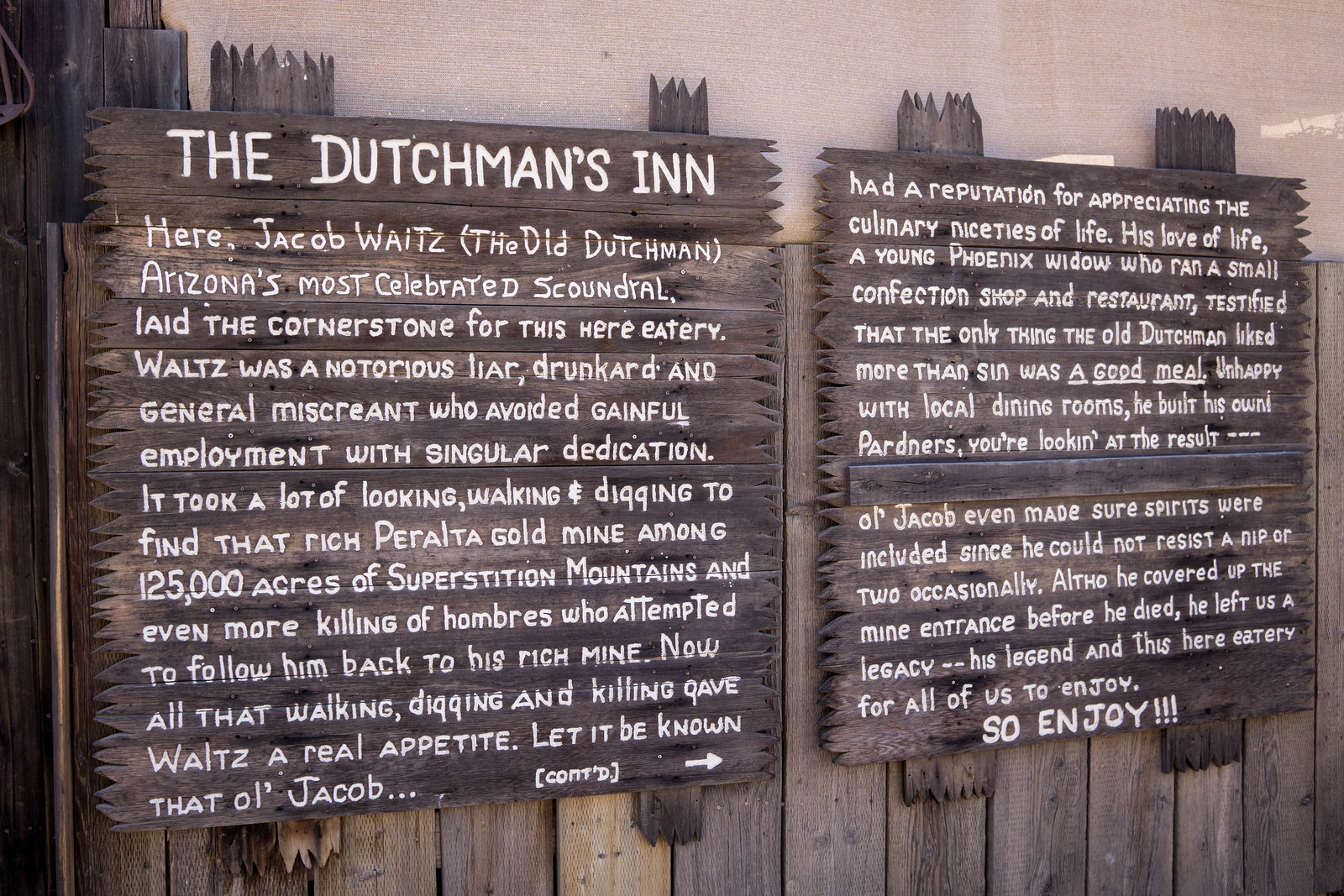In this black-and-white landscape-oriented photograph, two wooden signs are prominently displayed in front of a beige wall. The signs, marked with rugged, zigzag edges and mounted on vertical wooden posts with matching cut edges, are adorned with handwritten white text. The left sign bears the heading "THE DUTCHMAN'S INN," indicating it is for a restaurant or inn. Below the title, and continuing onto the adjacent sign to the right, is a detailed narrative about Jacob Waltz, also known as "The Old Dutchman." 

The text describes Jacob Waltz as "Arizona's most celebrated scoundrel," a notorious liar, drunkard, and generally unscrupulous character who steadfastly avoided gainful employment. Waltz famously searched through the 125,000 acres of the Superstition Mountains to locate the rich Peralta gold mine, involving much walking, digging, and even the killing of those who attempted to follow him.

This arduous quest is said to have given Waltz a considerable appetite, and his appreciation for fine dining is noted. A young Phoenix widow who owned a small confection shop and restaurant attested that Waltz loved a good meal almost as much as he loved sin. Dissatisfied with local dining options, Waltz built his own establishment, ensuring it included spirits, as he was known to indulge in naps. 

Despite hiding the mine's entrance before his death, Waltz left behind a legend and "this here eatery" for future generations to enjoy. The photograph captures not only these historical musings but also the rustic charm and historical insignificance of the signage.